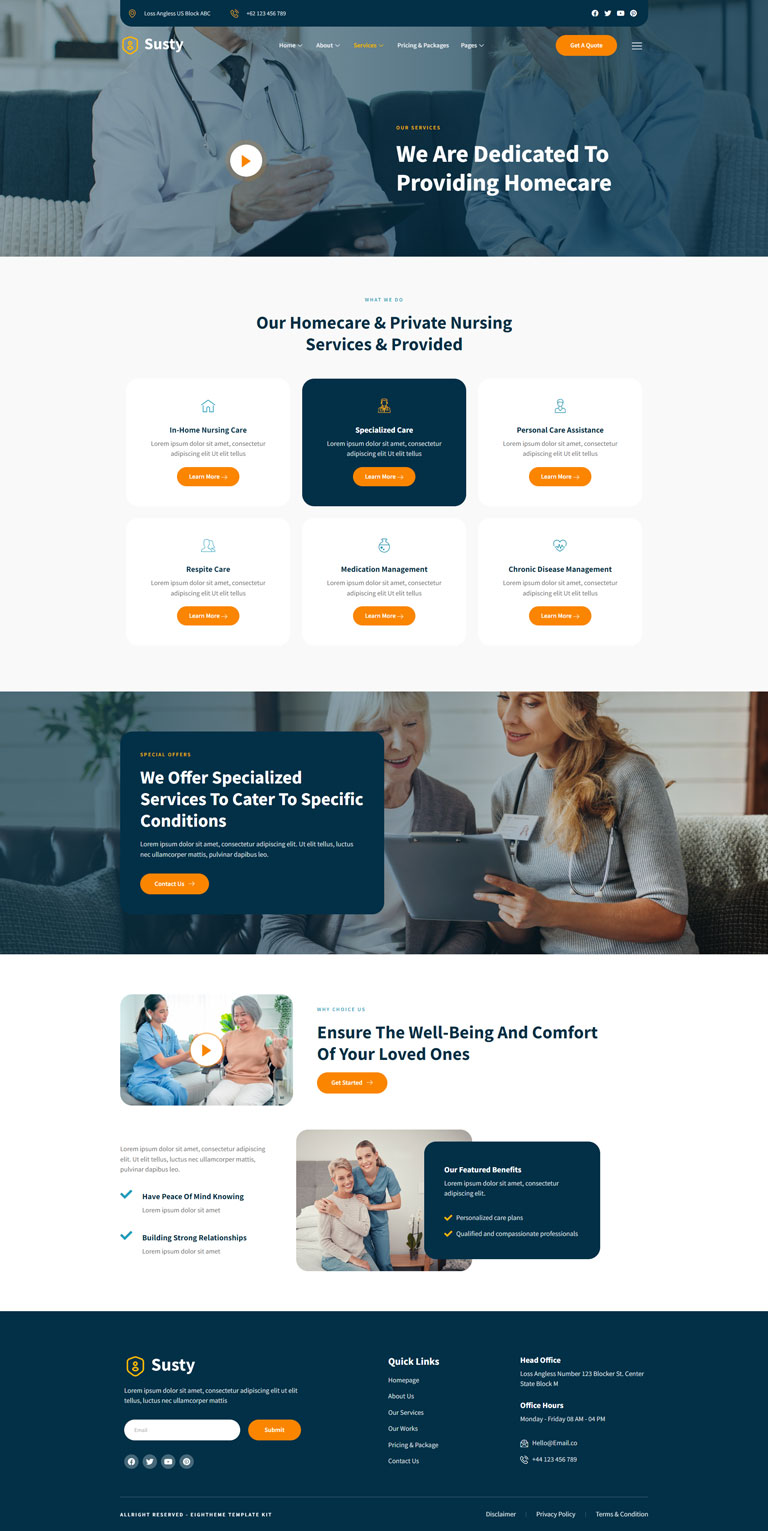In this image, the top section features a large black box with the name "Sonny" on the left side, accompanied by white text and an orange button that reads, "We are dedicated to providing home care." A white circle with an orange arrow points to the right, accentuating a doctor in the background, who is dressed in a white coat and wearing a stethoscope around his neck.

Beneath this, a blue box contains the message, "Our home care and private nursing service is provided." Below the blue box, there are five smaller white boxes, each pertaining to different in-home services, such as housekeepers and nursing assistants. Each service box includes an orange button at the bottom, with one box highlighted in black to draw special attention.

Further down, another image presents a black box with text stating, "We offer specialized services to cater to specific conditions," along with an orange button at the bottom. This part of the image shows two women engaged in conversation.

Following this, two additional pictures feature text emphasizing the importance of ensuring the well-being and comfort of loved ones, each accompanied by a little orange button. The concluding section of the image includes a larger black box at the bottom, containing a search box flanked by an orange button.